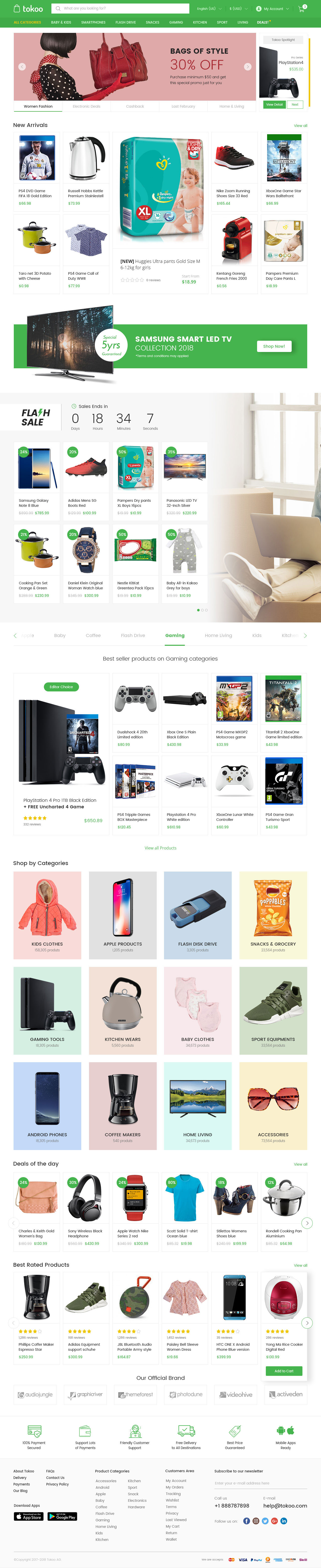This image appears to be a screenshot from an online store. At the very top, there's a medium green header followed by a pink navigation bar featuring a red purse with a "30% off" label. Below this, in the center, is an image of a pack of diapers. To the right, there's what looks like a teapot, some regular pots, and two other indistinguishable items.

Further down, another ad bar showcases a large flat-screen TV set against a green background. Beneath this, the store displays eight purchasable items, including pots, pans, a pack of diapers, and potentially some shoes. To the right of these items, there is an image of someone working at a desk.

Continuing down, there are options for purchasing gaming systems and controllers. Finally, the bottom section of the screenshot shows another set of eight items. Among them, some clothes are visible, although the rest of the items are unclear. This compact store layout seems designed to offer quick, diverse shopping options to its users.